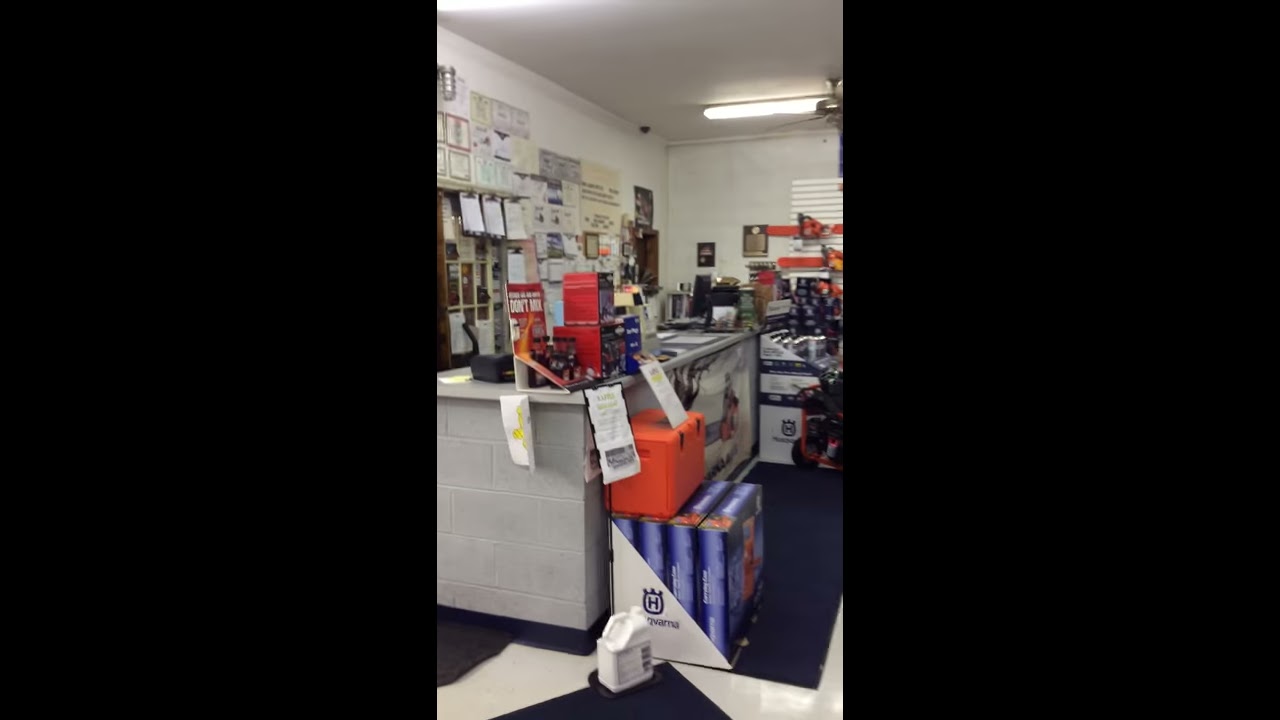The image depicts a cluttered indoor space that resembles a motor shop, hardware store, or office setting. At the center of the photo is a large stand or counter with various items scattered on and around it. In the foreground, the floor is covered with both hard tiles and different types of carpet. Four blue boxes and an orange box are positioned on the floor, although their contents are unclear. A white jug that looks like it might contain oil is also seen near these boxes. Above the counter, papers and packages are hanging, likely taped up. Additional boxes and papers are visible behind the desk area. The background includes walls with assorted items and a ceiling light. Various tools and equipment are spread around the scene, adding to the impression that this could be a space where motorized vehicles are serviced or items are sold. The predominant colors in the image are shades of blue, gray, black, white, orange, and red.